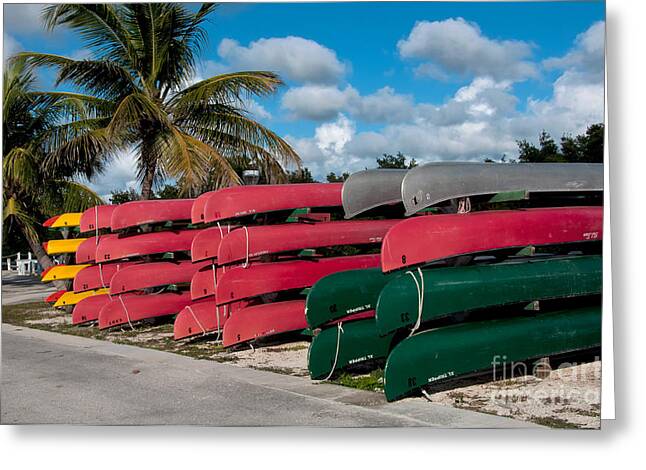The photograph features several stacks of canoes situated alongside a cement road, likely in a southern or tropical environment suggested by the presence of tall palm trees on the left. Each stack contains about four canoes, supported by a structure that secures them in place. In the foreground, there are four dark green canoes, two silver ones, and groups of yellow and white canoes. Most prominent are the numerous red canoes, intermingled throughout the stacks. Behind the canoes, the backdrop includes a blue sky dotted with puffy white and gray clouds and green vegetation. At the bottom right of the image, faint white text reads "Fine Art America," indicating the source of the image. The setting hints at an area where canoes can be rented, possibly near a marina or beach, given the sandy ground with patches of grass beneath the canoes. Ropes can be seen extending from the canoes, serving as a means to pull and maneuver them.